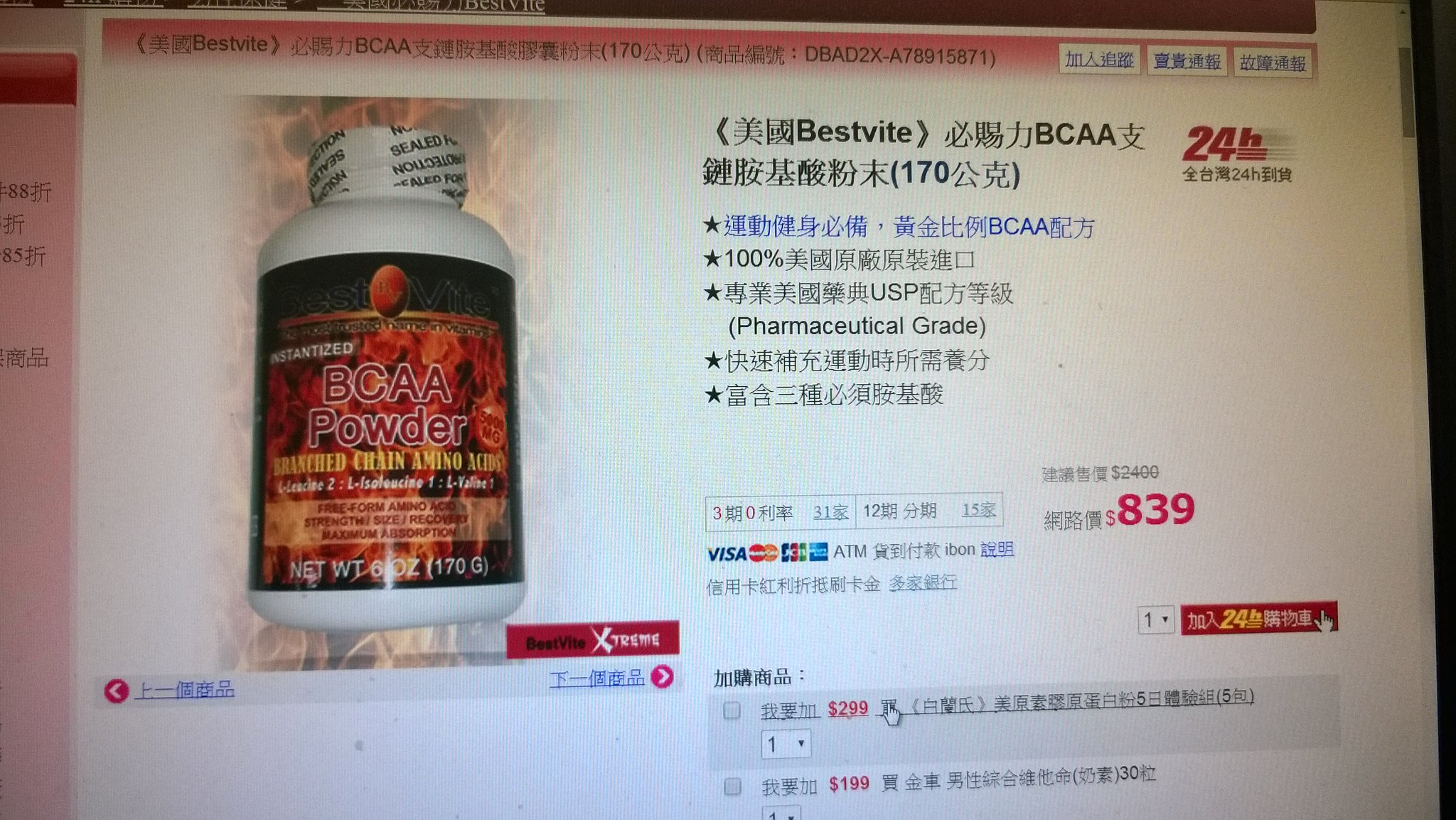The advertisement, likely a screenshot from a foreign website featuring predominantly Chinese or Japanese text, displays a clean, white background. Dominating the left side, a prominent white plastic bottle with a sealed top features the bold label "BCAA Powder". This label is eye-catching with its black border and red center, showcasing additional details like "net weight 6oz 170g". Above the product image, a thin black border aligns at the top, followed by a pinkish tab with white rectangles containing Asian characters. 

To the right of the bottle, several organized sections provide more product information: "Best Bite", "BCAA 170", and "USP Pharmaceutical Grade 100%" are notable English phrases among the primarily Asian text. Boldly highlighted in red text is "24H". Below, the purchase information includes recognizable symbols for Visa, MasterCard, and ATM, along with a price of ¥839. Lastly, a clickable icon resembling a finger indicates an option to proceed with the order, akin to online shopping platforms like Amazon.